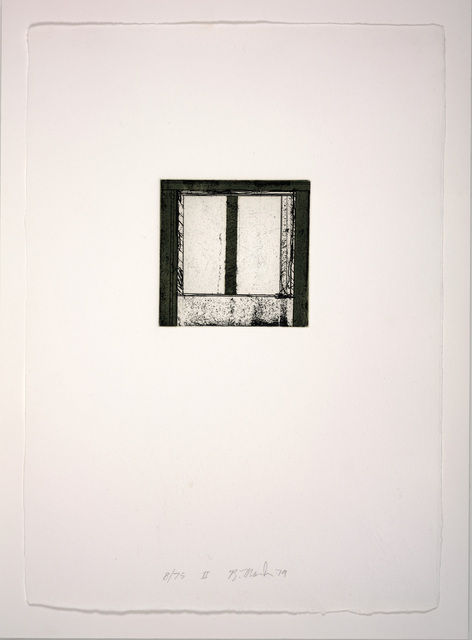This image captures a tall, rectangular photograph showcasing a hand-drawn illustration on a slightly tattered piece of paper against an off-white background. The paper's edges are uneven and ripped, suggesting it's been torn from a sketchbook or a similar source. At the bottom of the paper, small pencil writing, which appears to be a date and a signature, is visible.

Dominating the center of the composition is a window-like drawing, illustrated with what appears to be either black ink or pencil. The drawing features a square shape with a thick, solid black border along the left, top, and right edges. Inside the square, a thick vertical stripe bisects the image, possibly representing the window’s mullion. Near the bottom of this drawing is a horizontal, speckled rectangle, giving an impression of shadow or depth.

There are also smaller, straight, thin black lines inside the window frame, but they're irregular in placement, contributing to an abstract, somewhat un-uniform aesthetic. Along the bottom of the window, the speckled area, giving a slightly shadowy and textured appearance, provides further depth and intrigue to the simple yet evocative sketch.